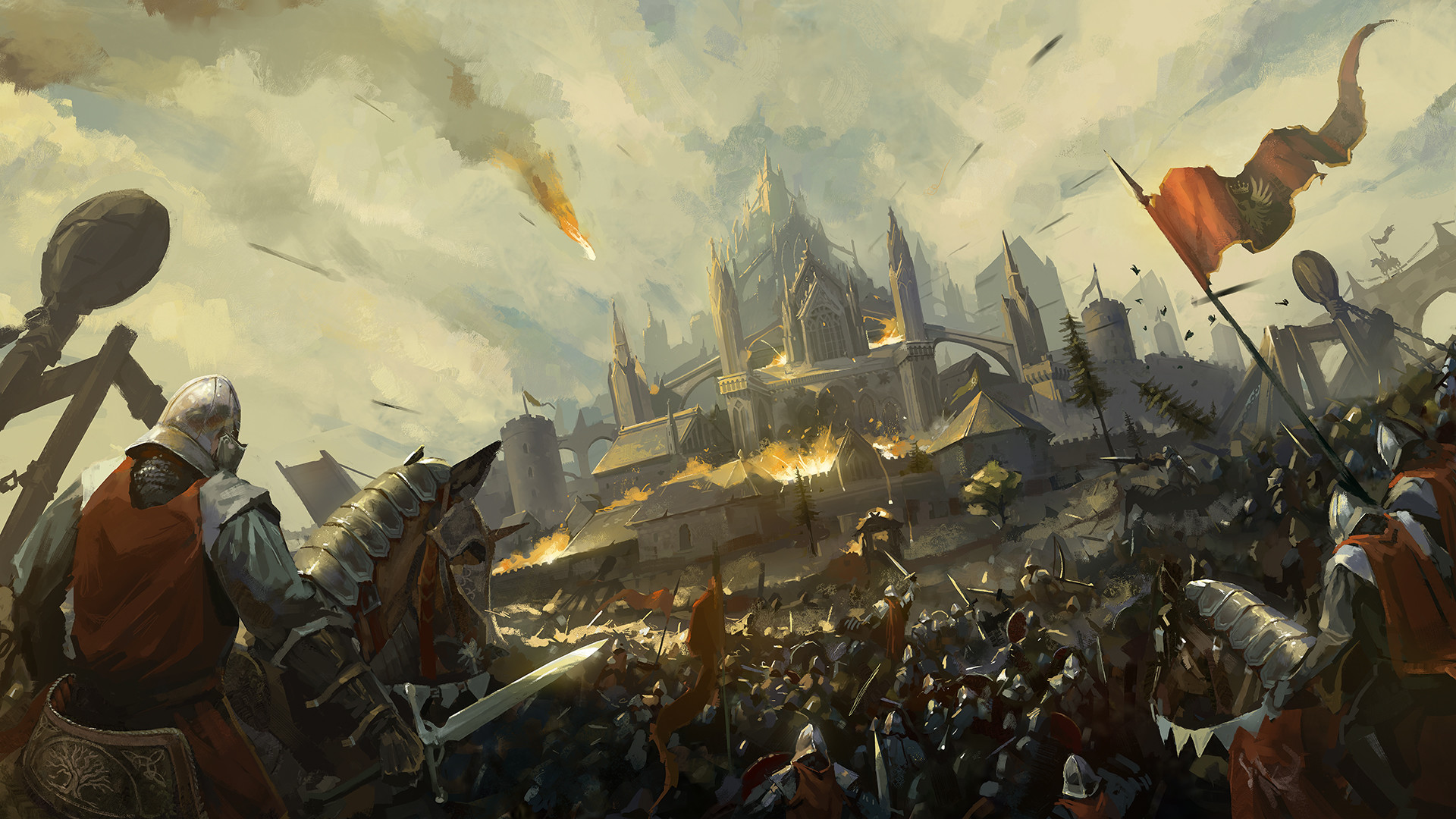The digital artwork depicts an intense siege on a large, multi-layered castle reminiscent of scenes from "The Lord of the Rings: The Return of the King." The structure features four distinct layers leading up to the top. In the foreground, buildings are engulfed in flames as knights donning grey armor and red garments lead the assault. The attacking forces utilize trebuchets and ride war horses, also adorned in red. Flags bearing eagle emblems flutter among the besieging troops, heightening the sense of epic battle.